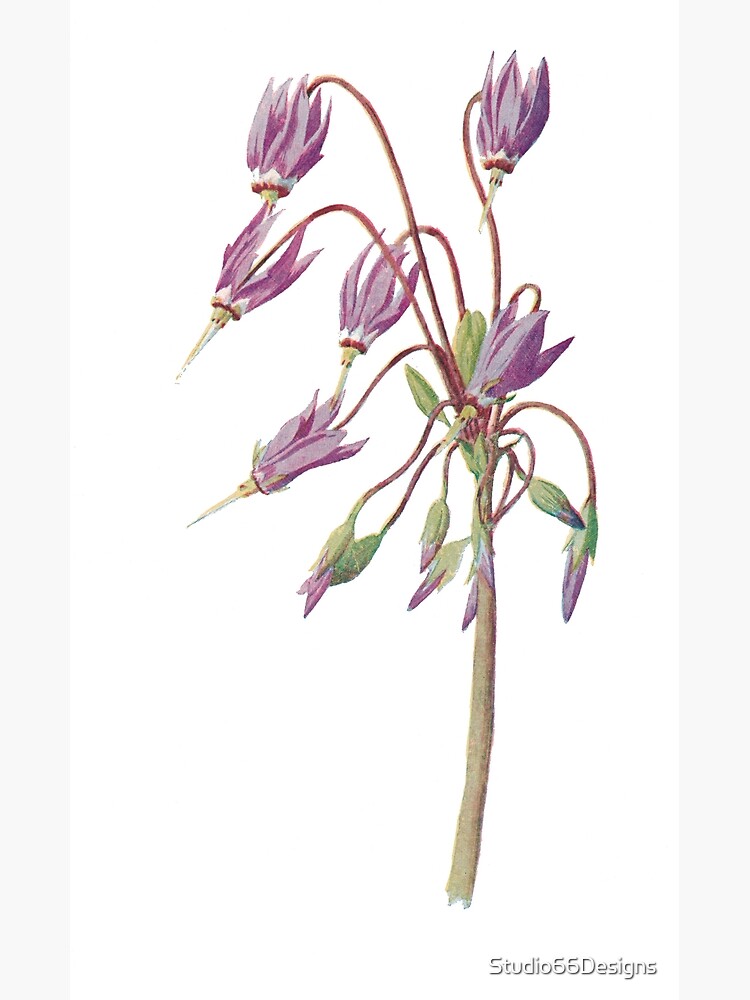This detailed watercolor painting, set against a white canvas, depicts a lilac to light purple flower with intricate elements. Rising vertically, the main stem is a beige to brown tone, leafless and sturdy. It branches into thinner, purple-hued offshoots that extend in various directions. Culminating in a vibrant and lively cluster, these offshoots bear purple flowers with distinct white and yellow beak-like centers. Some flowers are in full bloom with their delicate petals spread wide, while others remain in tight, green buds, waiting to unfurl. The artwork meticulously captures the contrast between the thin yet sturdy stems and the ethereal beauty of the flowers. In the bottom right corner, a watermark reads "Studio 55 Designs," marking the piece's creative origin.